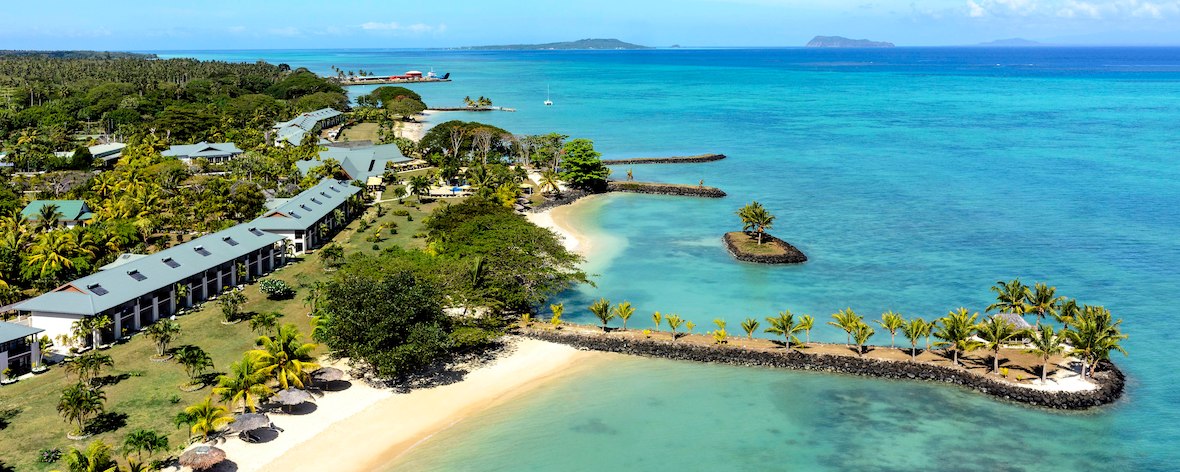This aerial photograph captures a breathtaking coastal scene where a beach resort blends seamlessly into its natural surroundings. The bright side of the image showcases an expansive ocean, transitioning from a dark blue hue in the far distance to a lighter, crystalline blue near the shore, where the white sands beneath the water become visible. Scattered around are clumps of dark gray rocks that add texture to the serene waters.

A prominent feature is a man-made dirt outcropping extending into the water, ending in a round cul-de-sac shape. Lined with multiple palm trees, this outcropping hosts a small bungalow, enhancing the tropical ambiance. Below this outcropping, the sandy beach stretches across the left side, where the dry sands are a pristine white that turn tan when wet. Beach umbrellas are strategically placed at intervals, offering shade to guests.

Behind the beach lies a well-manicured, flat green lawn, complementing the backdrop of a tall, long building with low-profile structures featuring multiple roof windows. The resort area is framed with lush green trees, further enhancing the idyllic setting. In the distance, small hills rise in gray against the horizon, adding depth and a sense of seclusion to the resort's picturesque environment. This photograph masterfully captures the essence of a tropical retreat, blending natural beauty with subtle human interventions.